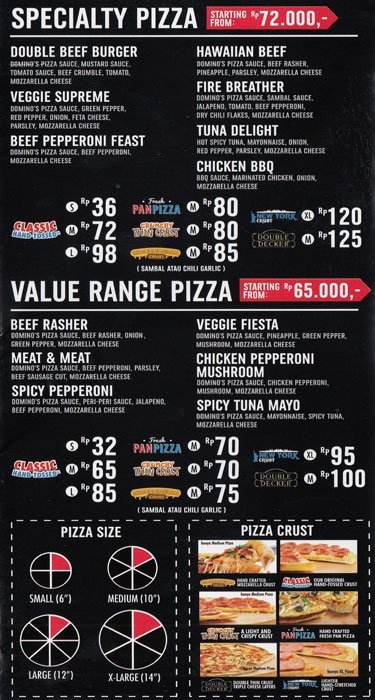This image is an advertisement poster for a specialty pizza establishment. The background is predominantly black, accentuating the various vibrant details. 

At the top section of the poster, there is a bold red banner on a black background, featuring the text "Specialty Pizza starting from 72,000", which is not in dollars. Next to it in white letters, different specialty pizza variations are listed such as Double Beef Burger, Veggie Supreme, Beef Pepperoni Feast, Hawaiian Beef, Fire Breather, Tuna Delight, and Chicken Barbecue. Each variation includes prices for various types of meals like pan pizza, classic, and New York crust. 

The center segment of the advertisement highlights "Value Range Pizza" starting from 65,000, with options like Beef Rasher, Meat and Meat, Spicy Pepperoni, Veggie Fiesta, Chicken Pepperoni Mushroom, and Spicy Tuna Mayo. Ingredients for each type are detailed underneath the options. 

The bottom part of the poster provides a comprehensive guide to pizza sizes and types of crusts available. On the left, a panel labeled "Pizza Size" in white lettering on a black background illustrates small, medium, large, and extra-large sizes. Adjacent to this, on the right, another panel labeled "Pizza Crust" displays actual images of the different types of crusts offered. Moreover, additional details about pizza categories like classic, hand-tossed, pan pizza, and New York crust with their corresponding prices are presented.

Overall, the poster is dense with information and images, structured to provide a thorough overview of the pizza shop's offerings, geared towards enticing potential customers with its detailed visuals and appealing variety.